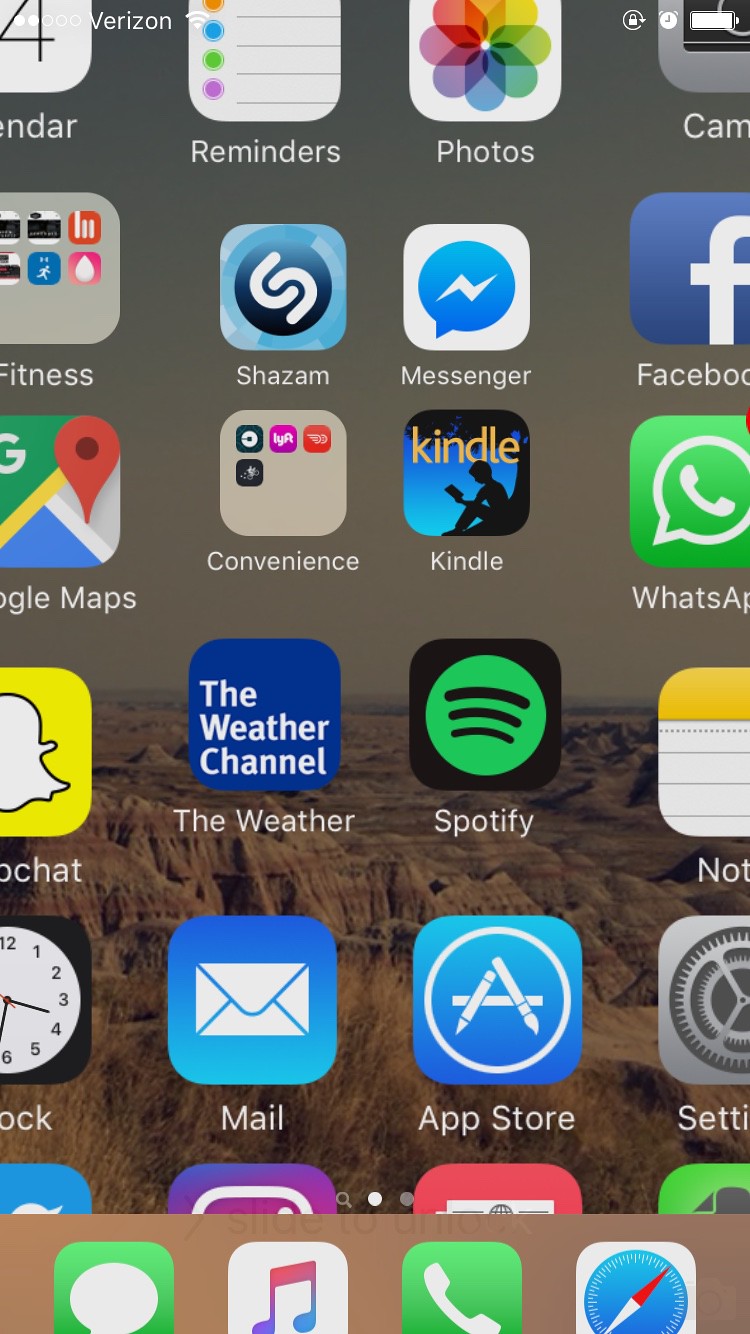A cropped screenshot of an Apple iPhone is on display, showcasing a vibrant Grand Canyon wallpaper. The intricate rock formations of the canyon serve as the backdrop. The home screen is populated with an array of apps, though some are partially cut off due to the cropped nature of the image. Visible apps include Calendar, Reminders, Photos, Camera, various fitness apps, Shazam, Messenger, Facebook, WhatsApp, and Kindle. In addition, a folder labeled 'Convenience' is discernible, housing apps like Uber, Lyft, and Postmates. Other recognizable apps include Google Maps, Snapchat, The Weather Channel, Spotify, Notes, App Store, Settings, Mail, and Clock.

The phone is identified as an Apple device running on the Verizon network, indicated by the signal strength icon in the top left corner. The status bar shows full Wi-Fi connectivity and a fully charged battery. At the bottom of the screen, the default dock features the Messages, Music, Phone, and Safari apps. The detailed, high-resolution image emphasizes the functionality and organization of the user's home screen amidst the stunning natural backdrop.